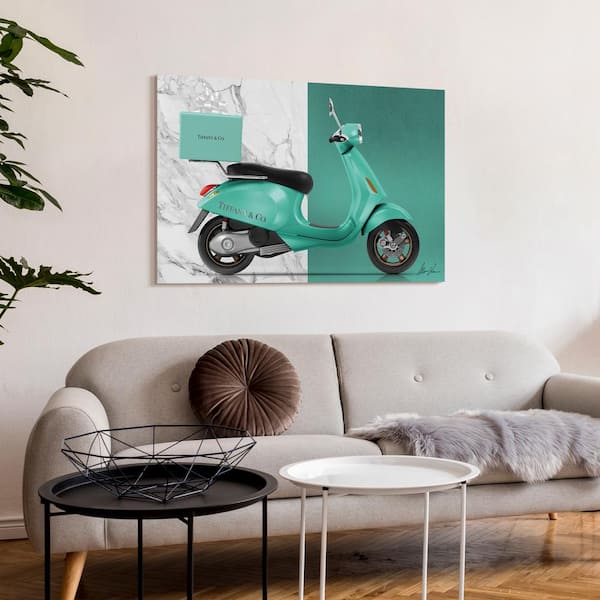This image captures a stylish, modern living room with parquet wood floors. Central to the scene is a low, creamy gray couch with wooden legs, positioned against a white wall. On the left cushion of the couch, a circular brown pillow is propped up, while the right cushion features a gray faux fur blanket. 

In the foreground, two small, round tables with skinny metal legs are placed side-by-side in front of the couch. The table on the left is black and has an open wireframe bowl, while the table on the right is yellow. 

Dominating the wall above the couch is a large, framed artwork of a side-view Tiffany Blue Vespa scooter. The scooter, which has a Tiffany & Co. logo on its back fender and a Tiffany box perched on its rear rack, is set against a uniquely split background—one half is Tiffany Blue, and the other is white and gray marble. 

A few green leaves of a tall house plant peek into the scene from the left side of the image, adding a touch of nature to the modern decor.